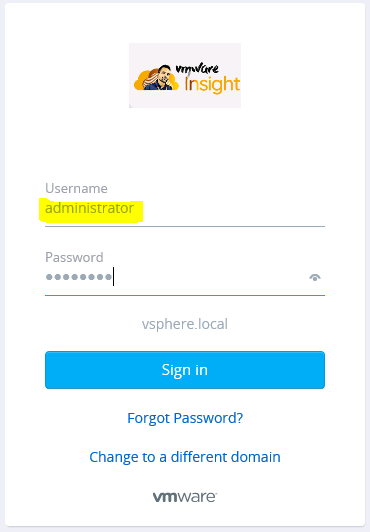This screen capture displays a detailed login screen. The focal point is a white box outlined by a thin gray trim. At the top of the box is a white square containing an illustrated image of a light-skinned man with black hair and facial hair, dressed in a blue shirt. Behind him is an orange bubble featuring a white and orange clothing object near his head.

Beneath this illustration is a section with black text where part of it appears to read "care" followed by the phrase "an orange insight" in orange font. The login section consists of two gray input lines. The first line is labeled "Username" with "administrator" entered, highlighted in yellow. The second line is labeled "Password," accompanied by placeholder circles and a black blinking cursor. An eye icon is positioned within this password field.

Below the fields is a blue line, underneath which appears the text "vsphere.local" in gray. The bottom of the box features a blue button labeled "Sign In" in white text. Adjacent to this button are two blue links: one stating "Forgot Password" and the other "Change to a different domain." At the very bottom of the screen, the text "VMware" is displayed in gray, concluding the screen's contents.